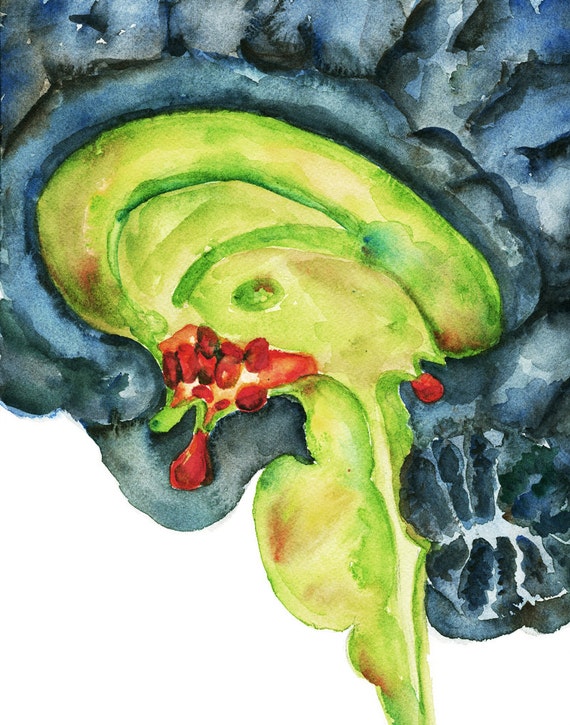This artwork is an abstract watercolor painting of a brain meticulously cut in half, emphasizing the amygdala, brain stem, and pituitary gland. The outer brain structure is rendered in a deep bluish-black, capturing its complex folds and crevices, while the central areas of interest are highlighted in various shades of green. Specifically, the amygdala and brain stem stand out in a vibrant grass green that draws the viewer’s eye.

In stark contrast to the dominant blue hues, the painting incorporates striking red details: berry-like blobs and drips accentuating the edges of the pituitary gland where it interfaces with the brain matter. These red elements likely denote significant aspects of the brain's anatomy or functions, adding a layer of depth and intrigue to the composition.

The background is a chaotic yet harmonious blend of grayish-blue watercolor blobs, creating a mottled backdrop that contrasts with the organized complexity of the brain. The lower left-hand corner remains pristinely white, highlighting the intensity and focus of the brain's depiction.

Adding to the artwork’s abstract nature, one can discern facial features within the brain's image—a central green dot resembling an eye, an arch similar to an eyebrow, and a green extension that could be interpreted as a nose. These elements, coupled with the red drips, suggest an abstract face akin to Picasso’s style, contributing to the multifaceted interpretation of the piece.

Overall, the painting cleverly merges anatomical precision with abstract creativity, transforming the brain into a surreal and captivating piece of art.